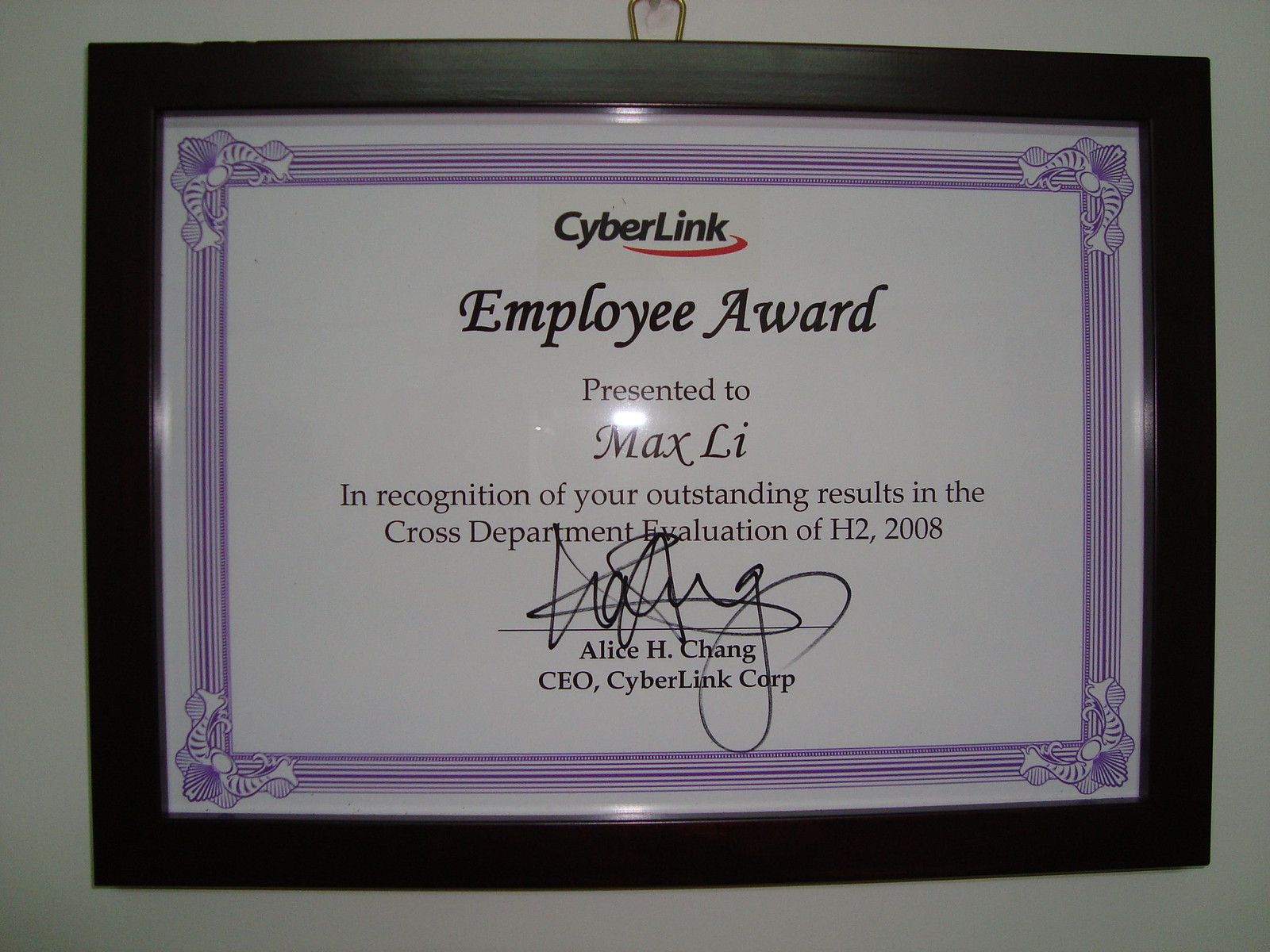The image shows a framed award with a glossy black, horizontally oriented 8x10 frame, hanging on a white wall. Inside the frame, the award is printed on white paper and bordered by a decorative purplish design featuring ornate scrollwork at each corner. At the top of the award, in black text, it reads "CyberLink," accompanied by a red logo below that runs from the letter 'E' to around the 'K.' Beneath this, in large black print, it states "Employee Award," followed by "presented to Max Lee." The subsequent line reads, "In recognition of your outstanding results in the cross-department evaluation of H2 2008." Lower on the paper, there is a large, scribbled signature, under which is printed "Alice H. Chang, CEO, CyberLink Corp." The image also captures the reflection of a light bulb on the glossy frame, indicating that the photo was taken with a flash or under strong lighting.